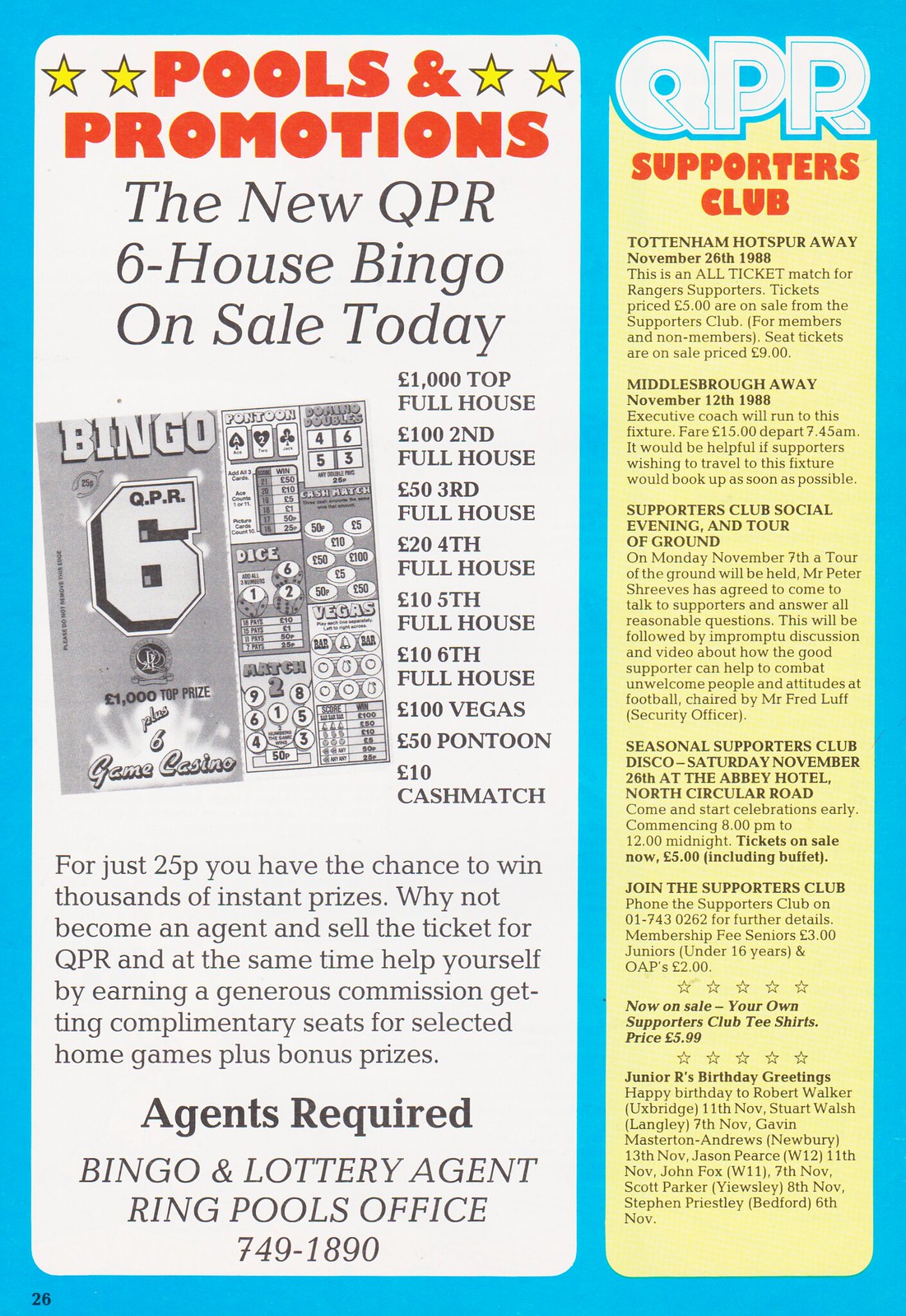The promotional flyer features a vibrant blue background with distinct white and yellow vertical sections. On the left side, the white section prominently displays the header "Pools and Promotions" in red, flanked by two yellow stars on either side. Below this, in black text, it advertises the new QPR Six House Bingo on sale today, with prizes listed as follows: £1,000 for the top full house, £100 for the second full house, £50 for the third full house, £20 for the fourth full house, £10 for both the fifth and sixth full houses, £100 for Vegas, £50 for Pontoon, and £10 for cash match. Additionally, there is an image of a bingo card. Information encouraging people to become agents and sell tickets for QPR appears in gray text, stating the benefits such as earning a generous commission, complimentary seats at selected home games, and bonus prizes. Agents are required, and those interested should contact the Pools Office at 749-1890. The yellow section on the right highlights QPR Supporters Club activities. At the top, in big white letters, it says "QPR," followed by "Supporters Club" in red. The section lists details about upcoming events like the Tottenham Hotspur and Middlesbrough away matches, Supporters Club social evenings and tours, the seasonal disco, and opportunities to join the Supporters Club. It also promotes the sale of Supporters Club t-shirts at £5.99 and features a section at the bottom for Junior R's birthday greetings. The page number 26 is noted in black in the bottom left corner.